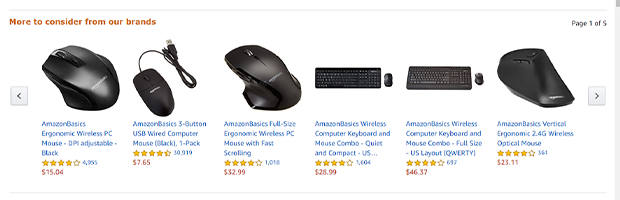The image features a clean white background accented with a light blue line running along the top, right side, and bottom. Prominently displayed at the top in red text is the phrase, "More to consider from our brands." On the left side of the image, there's a small blue box with a left arrow icon. The main focus is several computer peripherals with their prices listed. 

- A blue mouse priced at $15.04.
- Another mouse, presumably also blue, priced at $7.65, which is a wired model.
- A third mouse priced at $32.95.
- A keyboard priced at $28.99.
- Another keyboard priced at $46.37.
- A wireless optical mouse priced at $21.11.

The lower right corner of the image shows a small gray box with a right arrow, indicating navigation to the next page, which is identified as page 105. The overall visual suggests options for new mice or keyboards available for purchase.